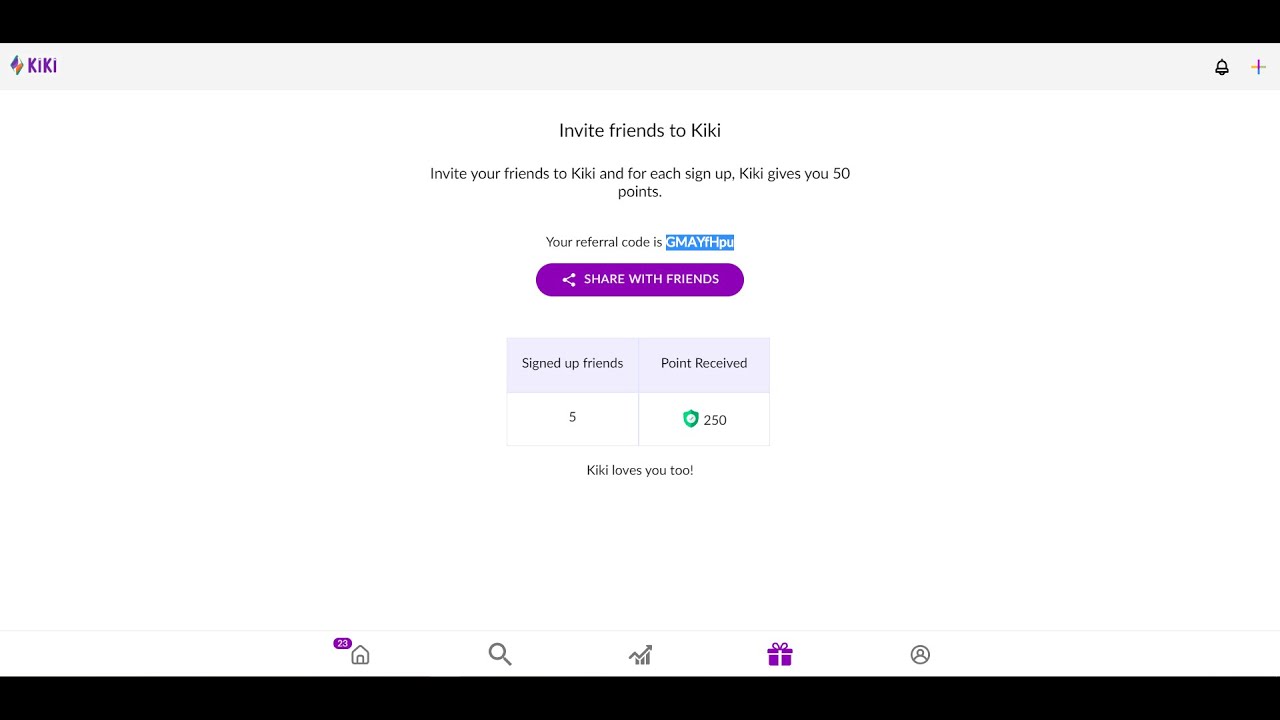The web page for the site Kiki is structured and colorful, with specific sections designed for user interactions and information display. 

At the very top of the page, a black bar stretches across the screen, providing a strong, sleek header. Directly below this, a white bar prominently features the Kiki logo, which is purple and accompanied by a small, flag-like or diamond-shaped icon to its right. The name "Kiki" is also displayed in purple text. Further to the right of the logo, there are notification and add buttons, symbolized by a bell icon and a plus sign respectively.

The main section below this header comprises mainly white and grey backgrounds. The first element you encounter here is an invitation banner that encourages users to invite friends to Kiki, capitalizing the "K" in "Kiki" for emphasis. The subsequent text explains that inviting friends to Kiki grants users 50 points per sign-up, and it also displays the user’s unique referral code, "GMA…" which is highlighted in blue text for easy visibility. 

Beneath this, there is a share bar prompting users to "Share with Friends," presented on a white and purple button. Another call-to-action below allows users to sign up friends, awarding 250 points and the message "Kiki loves you too."

Towards the bottom of the page, there's a utility bar featuring several icons. From left to right, they include a home symbol, a pie chart indicating the number of messages received, a search icon, a statistics icon, the current page icon, and a profile icon. Finally, the entire layout is anchored by a black bar at the very bottom, maintaining a clean and organized aesthetic.